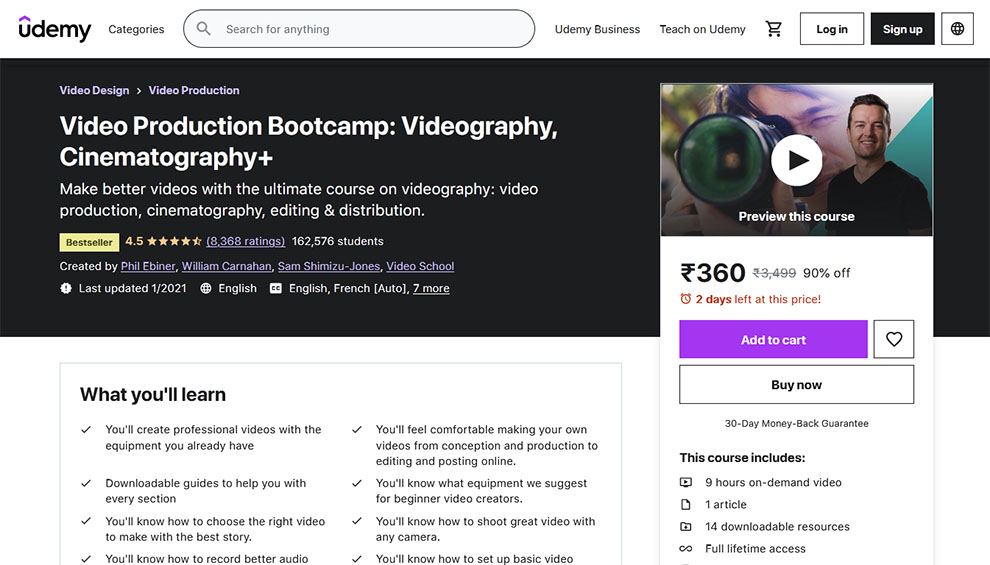The image depicts the homepage of the Udemy website. In the upper left-hand corner, the Udemy logo stands prominent, featuring an arrowhead above the letter "U". At the top of the webpage, a white navigation bar is visible, containing various elements from left to right: a "Categories" menu, a search bar labeled "Search for anything," followed by links to "Udemy Business" and "Teach on Udemy." To the far right, there are icons for the shopping cart, login, sign up, and an earth icon indicating language options.

Beneath the navigation bar, a promotional banner advertises a popular course titled "Video Production Bootcamp." The banner highlights that this comprehensive course covers videography, cinematography, video production, editing, and distribution. It is marked as a best seller with a rating of 4.5 stars and has enrolled 162,576 students, emphasizing its widespread acclaim and popularity.